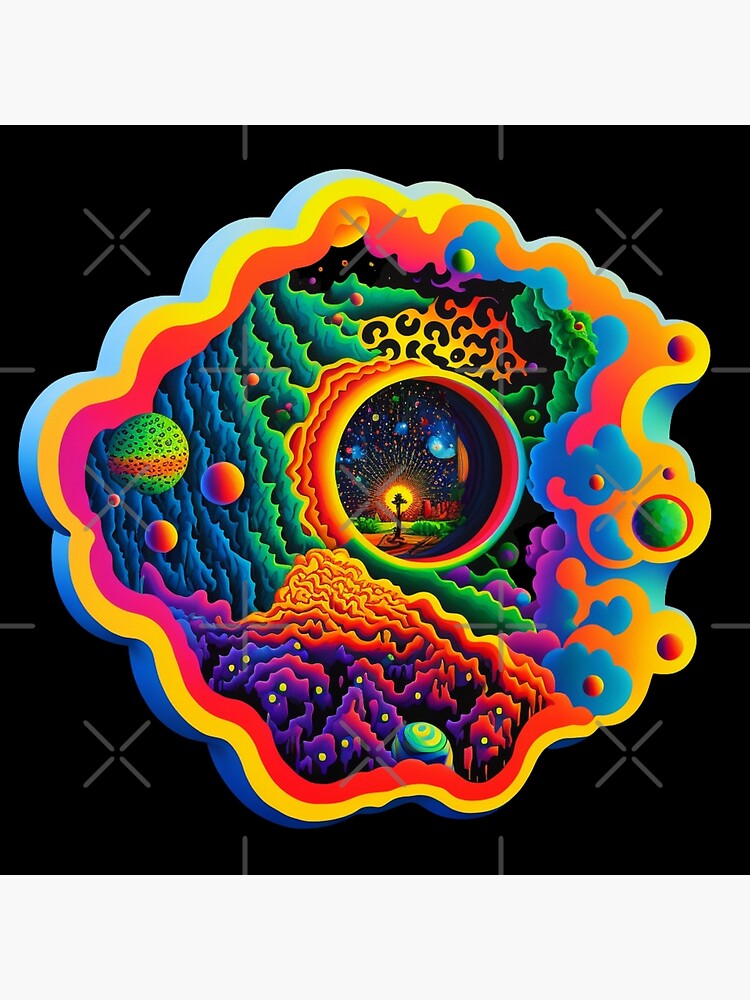This vertical rectangular image is an artist's drawing set against a black background with semi-transparent white X-shaped watermarks at each corner. Dominating the center is an irregular and vibrant, colorful figure. The outer edge of this shape starts as light blue at the top, deepening to darker blue at the bottom. Encircling this is a rim of yellow, bordered on the outside by a gradient of red transitioning to orange. Within this central figure, an intricate design of waves, lava, mountains, and flowing organic shapes, filled with vivid hues of greens, yellows, blues, reds, and purples, creates a dynamic impression of movement and depth. Near the center lies an off-center circle resembling a lens, containing an illuminated cross against a backdrop of what looks like a sunset on a grassy hill, transitioning into a night sky dotted with planets and stars. The overall piece evokes a psychedelic, trippy atmosphere rich with bright colors and intricate details.